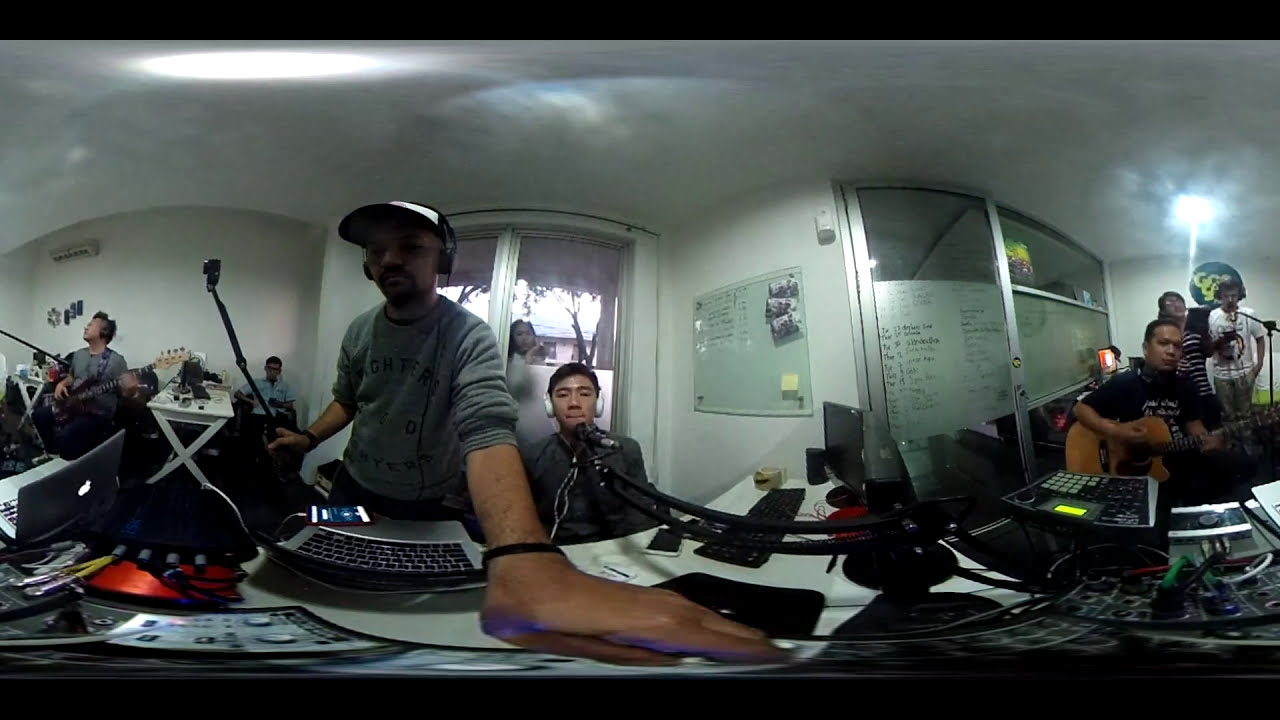This wide-angle, distorted photographic image captures an indoor music studio bustling with activity. Front and center, an Asian man is seated with headphones on, deeply engaged with the scene around him. To his left, another man in a baseball cap operates a control panel, while further left, a musician stands, playing the guitar and singing into a mounted microphone. To the right, under a wall-mounted bulletin board and some tech equipment, another seated Asian man strums a guitar. Behind him, a woman in a black and white striped dress studies a tablet, and a man in a white t-shirt with black markings, wearing headphones, talks into a microphone. The room features multiple walls, one plain white, one with open windows showing a gray sky, one adorned with a whiteboard, and the last with a sliding glass door. The walls and ceiling appear rounded due to the wide-angle lens. Additional tech equipment and laptops are scattered around, emphasizing the studio’s busy, music-oriented environment. Despite the many elements, no readable text is visible in the image.